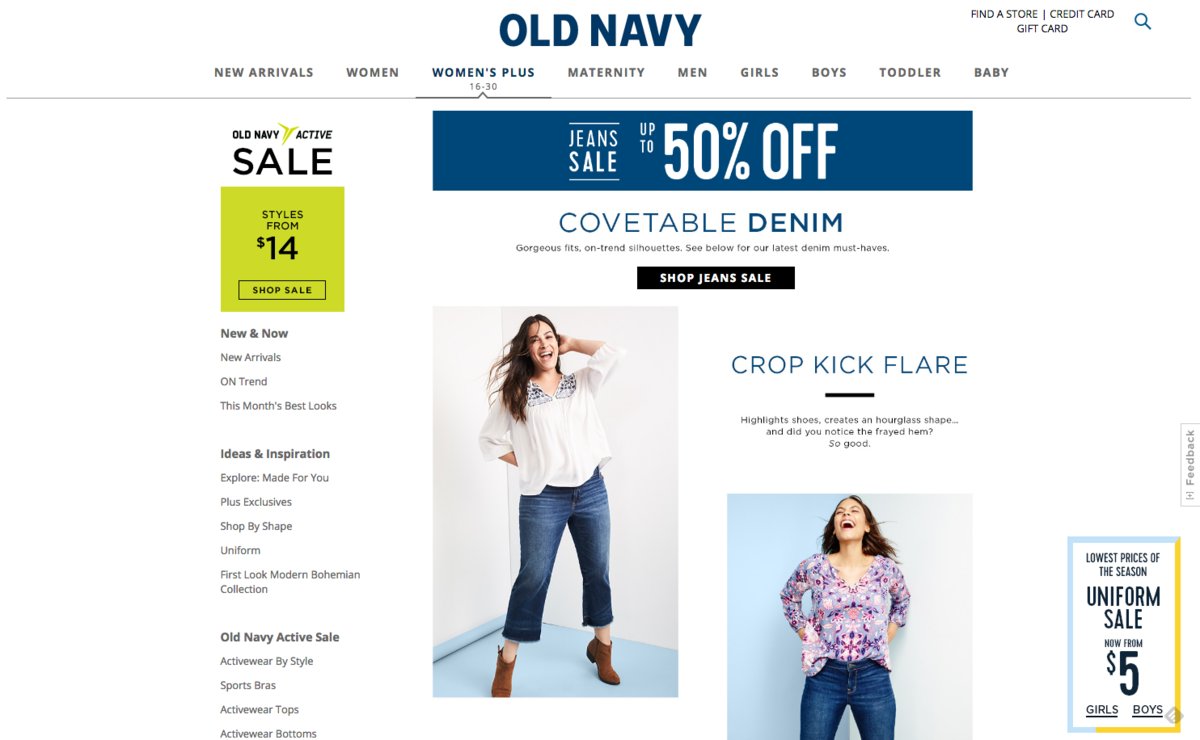Screenshot of the Old Navy Webpage: A detailed view of the Old Navy website showcases the store's offerings and navigation options. "Old Navy" is prominently displayed at the top center of the page. Users can easily access options to find a store, apply for a credit card, or purchase a gift card. The main menu includes categories such as New Arrivals, Women, Women's Plus (sizes 16 to 30), Maternity, Men, Girls, Boys, Toddler, and Baby.

A prominent advertisement highlights a sale on jeans with discounts up to 50% off, featuring catchy phrases like "Covetable denim, gorgeous fits, on-trend silhouettes." Below the ad, there's a call-to-action button inviting users to "Shop the Jeans Sale."

The section also includes two vibrant photographs of a model showcasing the jeans. In the first image, the model with long dark hair stands with her right hand on her hip and her left arm bent at the elbow, hand resting behind her head. She is dressed in a white embroidered elbow-length sleeved shirt, cropped blue jeans, and brown ankle boots, and is posed diagonally towards the right.

In the second photo, the same model faces straight ahead with her head tilted back and mouth open as if laughing. She is clad in a purple long-sleeve t-shirt and blue jeans, standing with her legs apart in a V-like pattern. The images highlight the stylish versatility of Old Navy's denim collection, enticing shoppers to explore the latest trends.